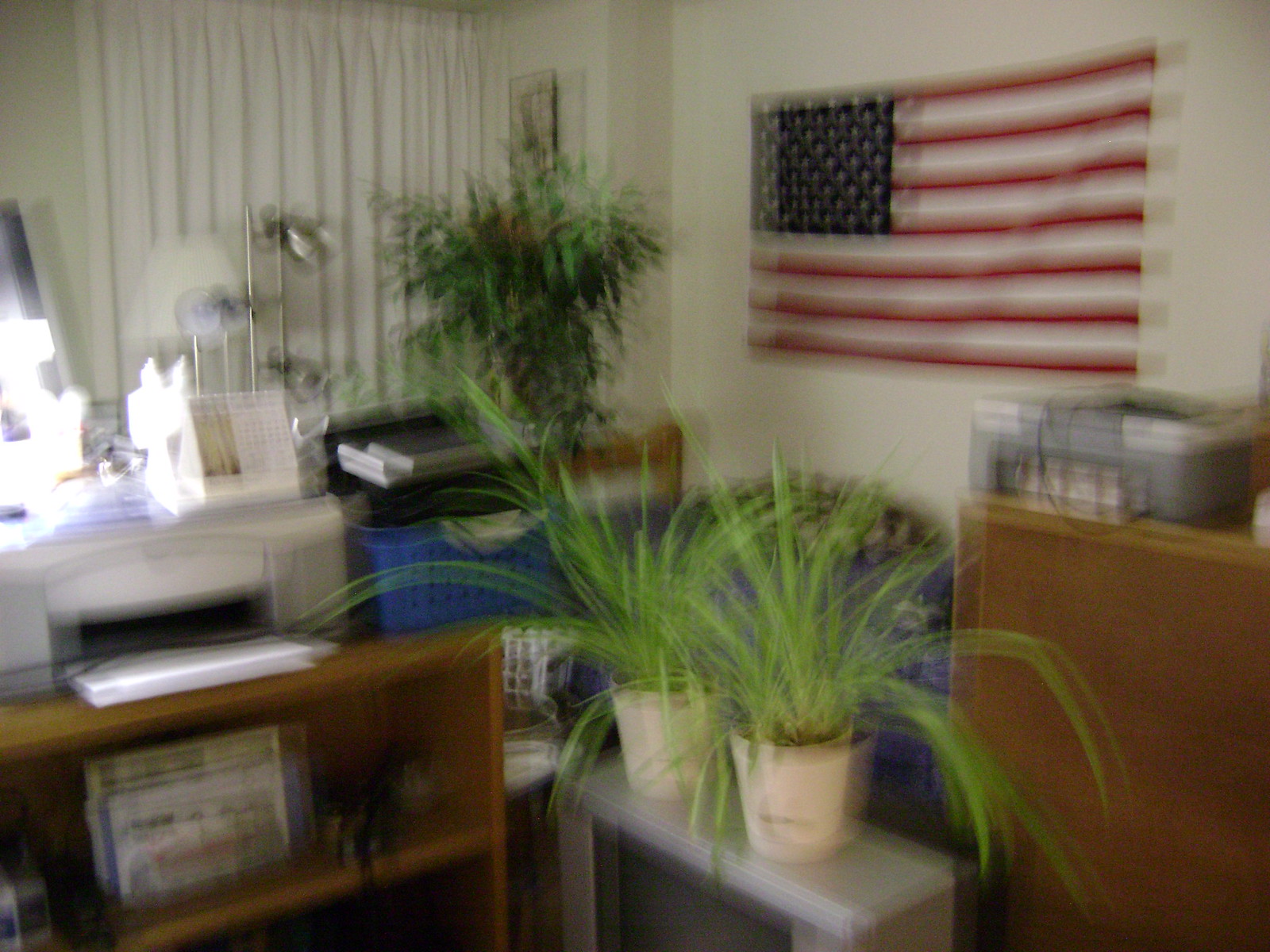The image is a color photograph, albeit slightly out of focus, depicting a corner of a room where two off-white or possibly beige walls intersect. Dominating the right side of the image, an American flag with red, white, and blue stripes hangs prominently. Below the flag, there's a piece of furniture, potentially a cabinet or table, with a gray object on top that resembles office equipment or an organizer. Adjacent to this is a smaller table hosting a couple of plants, contributing a touch of greenery to the scene.

A separate printer table is also visible, supporting a white printer, with various items tucked underneath it, suggesting a functional space. Additionally, a curtain can be seen draped along the other wall, further framing the room. Scattered around are a few more plants and a collection of items including at least two lamps—a white-shaded lamp and possibly a silver one—adding layers of detail and texture to the setting.